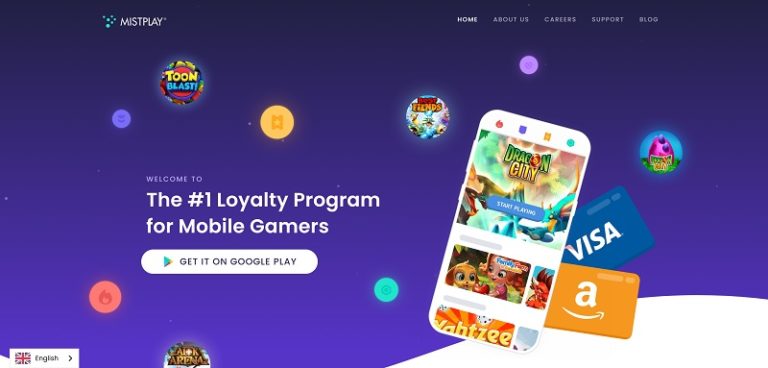The image features a website interface divided into two sections: the top half is a dark purplish-blue color, while the bottom half is solid white. In the top left corner, 'Missed Play' is prominently displayed. The top right corner boasts several navigation options including 'Home,' 'About Us,' 'Careers,' 'Support,' and 'Blog.'

Central to the design are several circles scattered across the blue area, with three large circles standing out among smaller ones. The first large circle shows "Tomb Blast," the second one highlights "Best Fiends," and the third features "Purple Egg" and "Merged Dragons."

In the middle of the composition is an image of a smartphone. On its screen, in a square area at the top, "Dragon City" is displayed alongside a button labeled "Start Playing." Beneath the phone are a series of small rectangular scenes from other games, partially obscured by Amazon and Visa gift cards, the left corners of which are tucked under the phone.

The bottom section welcomes viewers to "the number one loyalty program for mobile gamers" and encourages them to "Get it on Google Play." Various additional circles, differing in size, fill the remaining blue space, complementing the main elements of the image.